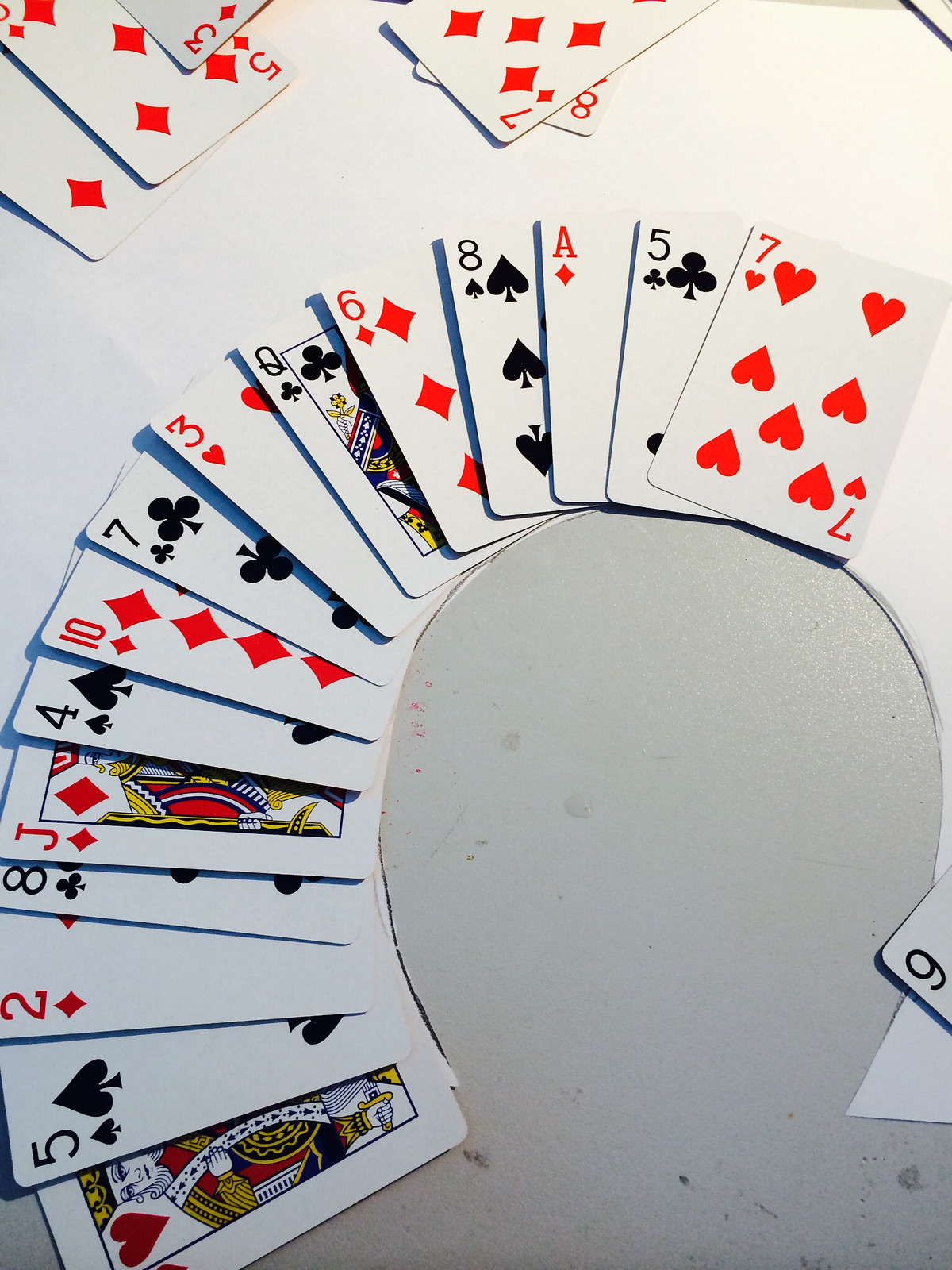A meticulously arranged, indoor color photograph looking down on a pristine white tabletop. Precisely fanned out across the lower left side of the table are 15 playing cards, all face-up, forming a diagonal curve that extends to the right edge. The sequence of cards displayed from bottom to top includes: the King of Hearts, the Five of Spades, the Two of Diamonds, the Eight of Clubs, the Jack of Diamonds, the Four of Spades, the Ten of Diamonds, the Seven of Clubs, the Three of Hearts, another Eight of Clubs, the Six of Diamonds, the Eight of Spades, the Ace of Diamonds, the Five of Clubs, and the Seven of Hearts.

In the upper left corner, two additional Diamond cards are partially visible, though their values are obscured. Centered towards the top edge of the frame, a Seven of Diamonds is prominently displayed, with an Eight of Diamonds peeking out from behind it. On the right side, part of a Nine of Diamonds is discernible.

A notable feature in the center of the table is a neatly cut gray circle, its exact purpose unknown, adding a curious element to the composition. The gray circle is more pronounced towards the bottom of the image, contrasting subtly with the white background. The illumination, coming from above, casts a soft light over the scene, making the top of the image appear brighter.

The arrangement of the cards suggests an intentional artistic design rather than a snapshot of a card game in progress. The cards, looking almost brand new, are methodically placed, hinting at the creation of a visually appealing poster or a similar creative project.